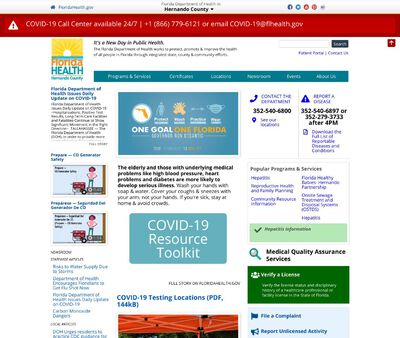The image is a small, square-shaped graphic with a primarily white background and vertical white borders on either side. Prominently featured at the top of the image is a bright red, thin, horizontal rectangular box. Inside this box, on the left side, is a white triangle with an exclamation point resembling an emoji. Next to this triangle, the white text reads, "COVID-19 Call Center available 24-7," followed by a phone number, likely 646-779-6121, or an email address, potentially COVID-19@health.gov.

Directly below the red box are various tabs and images. On the left, there is an image of a book placed beside a yellow flower, with the text "Florida Health" inside it. At the center, a larger blue rectangular section displays various icons, including a gun, a masked person, and other symbols. Beneath this section, bold black text is visible.

To the right, different contact resources such as phone numbers and email addresses are highlighted in blue. On the left side, additional black text can be seen. Towards the bottom left of the image, there are two smaller images of the same person, possibly holding a wagon. Finally, the bottom of the image features several blue links.